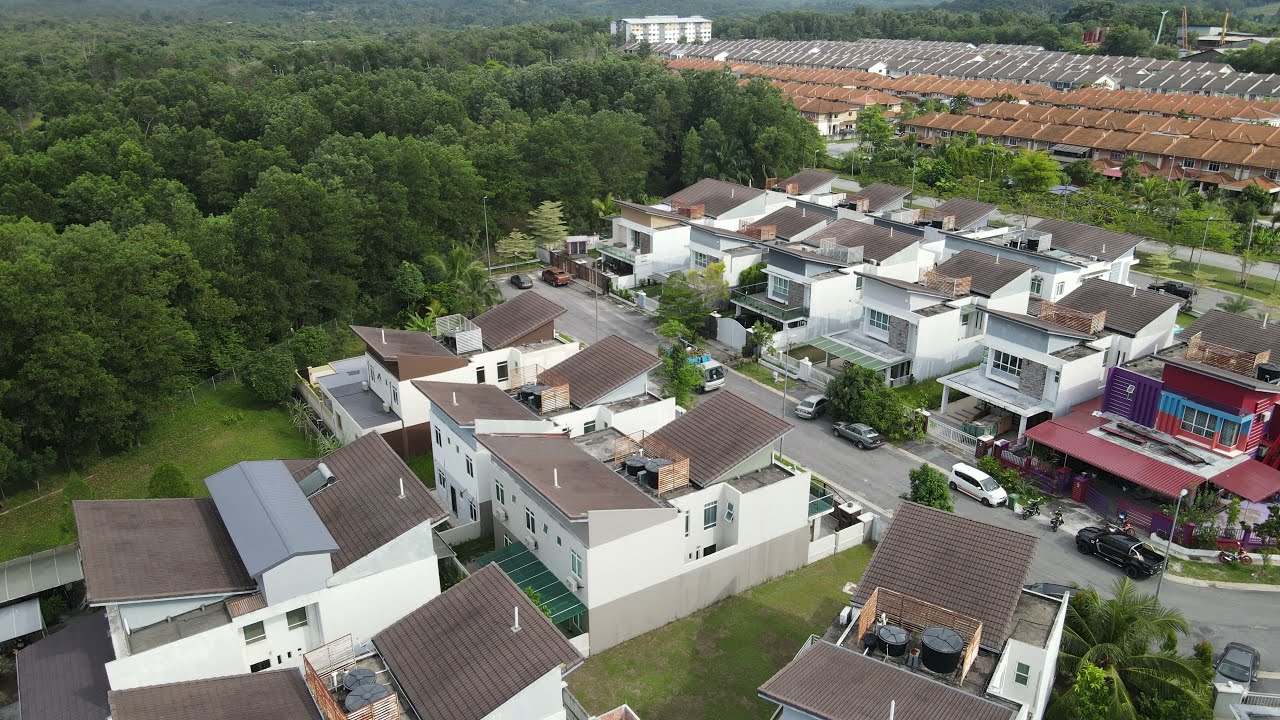This aerial daytime photograph captures a densely populated neighborhood with numerous houses aligned along intersecting streets. The front of the image showcases white, two-story townhouses with brown roofs, closely packed together, while the upper right portion reveals an extensive stretch of additional housing. These back rows transition to gray rooftops. A unique red and blue-striped building, potentially a restaurant, stands out on the far right side. A couple of cars are visible parked on the streets. Dominating the left half from the center to the lower edge, a dense forest of deciduous trees provides a stark contrast to the urban sprawl.